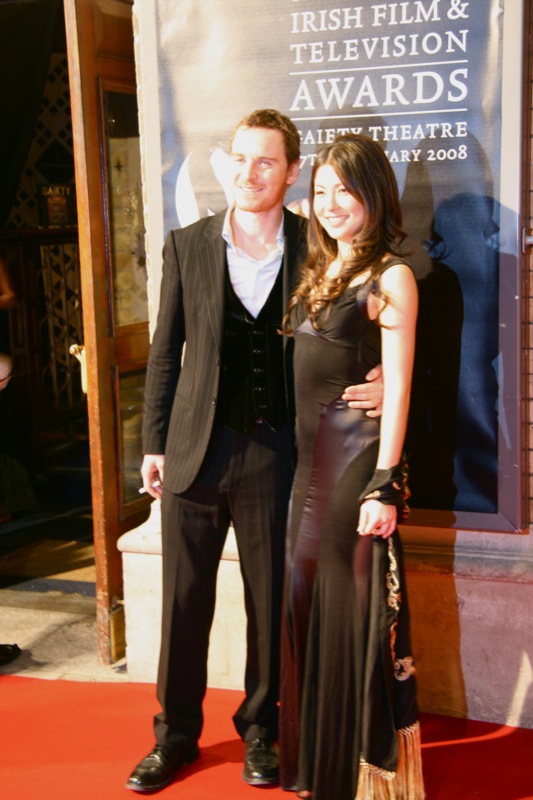This is an outdoor photo from the Irish Film and Television Awards 2008, possibly taken on January 7th in Ireland. The setting features a wooden, brown open door on the left, with a red carpet extending across the image. Two people are posing and smiling directly at the camera. The woman on the right is in a sleeveless black silk or satin dress, with a scarf wrapped around her left hand. She has long brown hair cascading past her shoulders. To her left stands a man in a dark pinstriped black suit, with a white shirt and a black under-jacket. He has close-cropped brown hair and his left arm seems to rest around the woman's waist. Behind them is a prominent poster for the Irish Film and Television Awards, adding to the event atmosphere. The lighting suggests the photo could have been taken in the late afternoon or early evening.